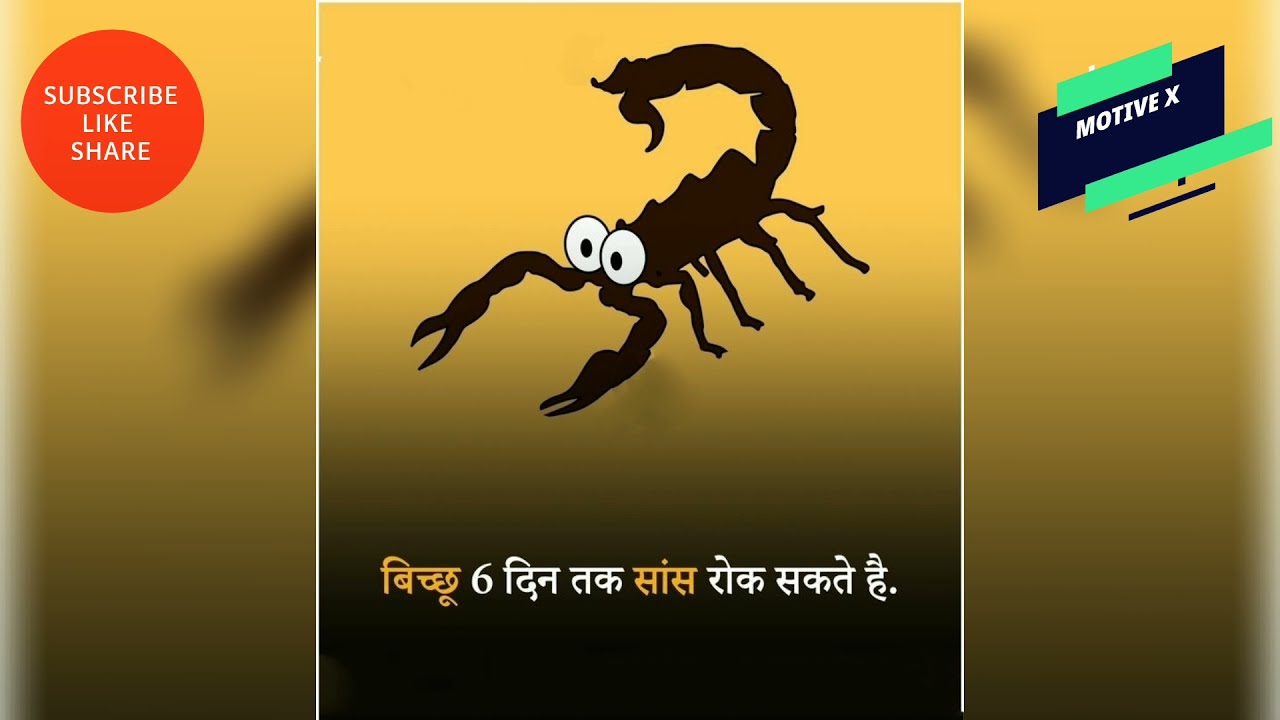The image features a visually striking graphic of a cartoon scorpion, depicted in shades of brown and black. The scorpion has large, googly white eyes with black pupils, giving it a whimsical appearance. The scorpion is a silhouette, facing slightly towards the bottom left corner. It is set against a vibrant yellow background that gradually fades to black at the bottom.

The image is framed by a white square border. In the top left corner, there is a prominent red circle with white text that reads "Subscribe, Like, Share." On the top right, a dark blue rectangle is prominently featured, decorated with light blue parallelograms, and contains the text "Motive X" in white.

At the bottom of the image, there is text in a different language, which appears to be written in Southeast Asian or Devanagari script, featuring both yellow and white characters. The writing is partly obscured and difficult to interpret. The overall design suggests that it might be an advertisement or a promotional graphic.